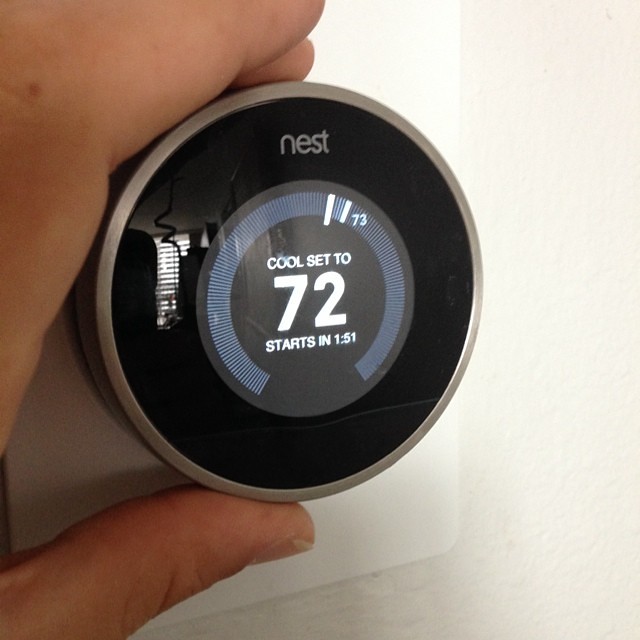The photograph displays a close-up view of a circular Nest thermostat, held by a person's left hand. The setting is against a white wooden surface that resembles a panel within a door or possibly a cubbyhole. The person's thumb is visible on the left side, while their index and middle fingers, shown from a profile view, are positioned from the center left to the top center of the image, gripping the outer edge of the thermostat.

The Nest thermostat itself is predominantly black with a sleek, possibly metallic, silver-edge design. At the top, the word "nest" is clearly displayed in gray letters at the 12 o'clock position. The device interface features an almost complete gray circular line, highlighting "73" in white at the 1 o'clock position. The central text on the screen reads, "cool set to 72, starts in 1 minute and 51 seconds." The black surface of the thermostat reflects a window with blinds, which appears on the left edge of the device, providing an additional visual element.